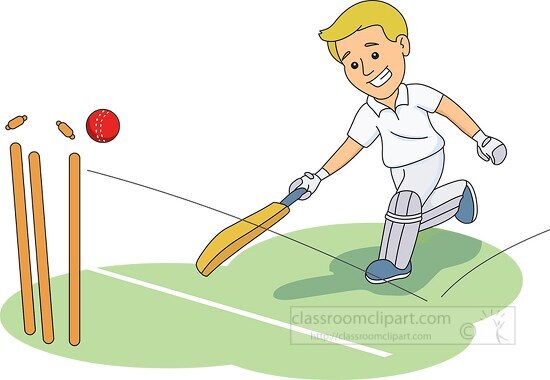The image is a digitally-created, cartoon-like illustration featuring a young Caucasian boy with blonde hair and black eyes, smiling as he engages in a game. He is dressed in a white short-sleeved, collared polo shirt and matching white pants, equipped with gray shin guards, blue shoes, and white gloves. He holds a scoop-like paddle in his right hand and is either about to catch or has just tossed a midair red ball. The scene includes three orangey-gold broomstick-like poles positioned where the ball appears to be bouncing upwards. Additionally, there are two smaller, hot dog-shaped objects in the air. The background consists of a green, bubbled-out area on the ground marked with white lines resembling those on a tennis court. The illustration includes motion lines indicating the ball's trajectory and a plain white background. In the bottom right corner, there is a watermark that reads "classroomclipart.com" along with a small, indistinct logo of a stick figure and a partially legible website.